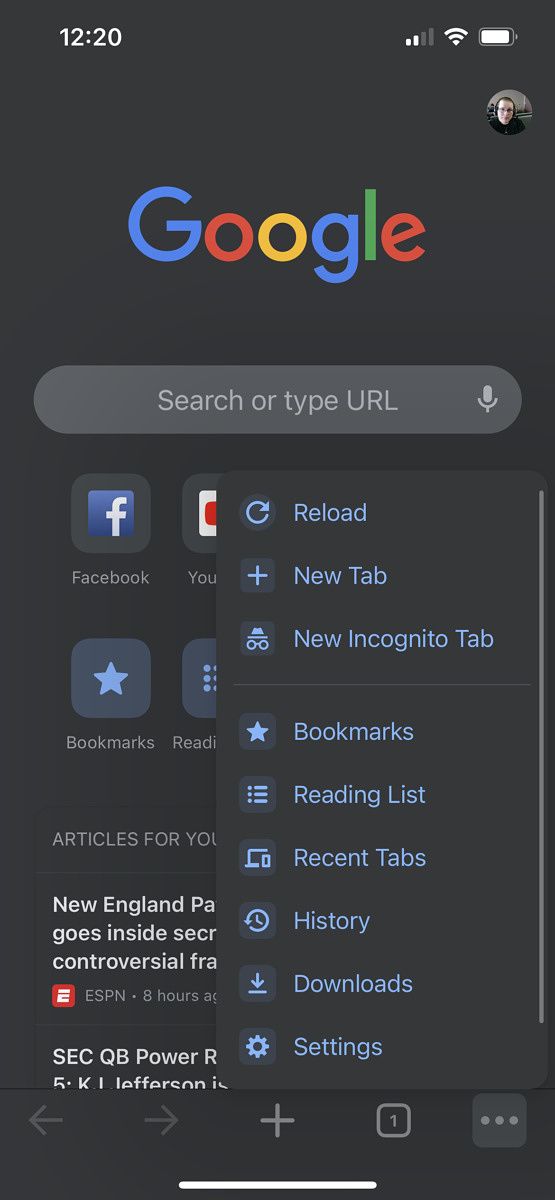The image is a screenshot taken from a mobile device, displaying the Google homepage. The background of the screen is a dark gray color, providing a sleek and modern look. At the top center of the screen, the iconic Google logo is prominently featured, with its letters colored individually in blue, red, yellow, blue, green, and red.

Below the Google logo lies a rectangular search bar, which occupies a central position on the screen. The search bar is light gray in color and has gently curved corners, giving it a smooth and approachable appearance.

On the right side, just below the search bar, there is a pop-up menu with a list of options, all written in blue. Each option is accompanied by a corresponding icon on its left side, making it easy to identify the function at a glance. The options, listed from top to bottom, are: 
1. Reload
2. New tab
3. New incognito tab
4. Bookmarks
5. Reading list
6. Recent tabs
7. History
8. Downloads
9. Settings

This detailed and organized menu provides quick access to various functionalities, enhancing the user experience on the mobile device.